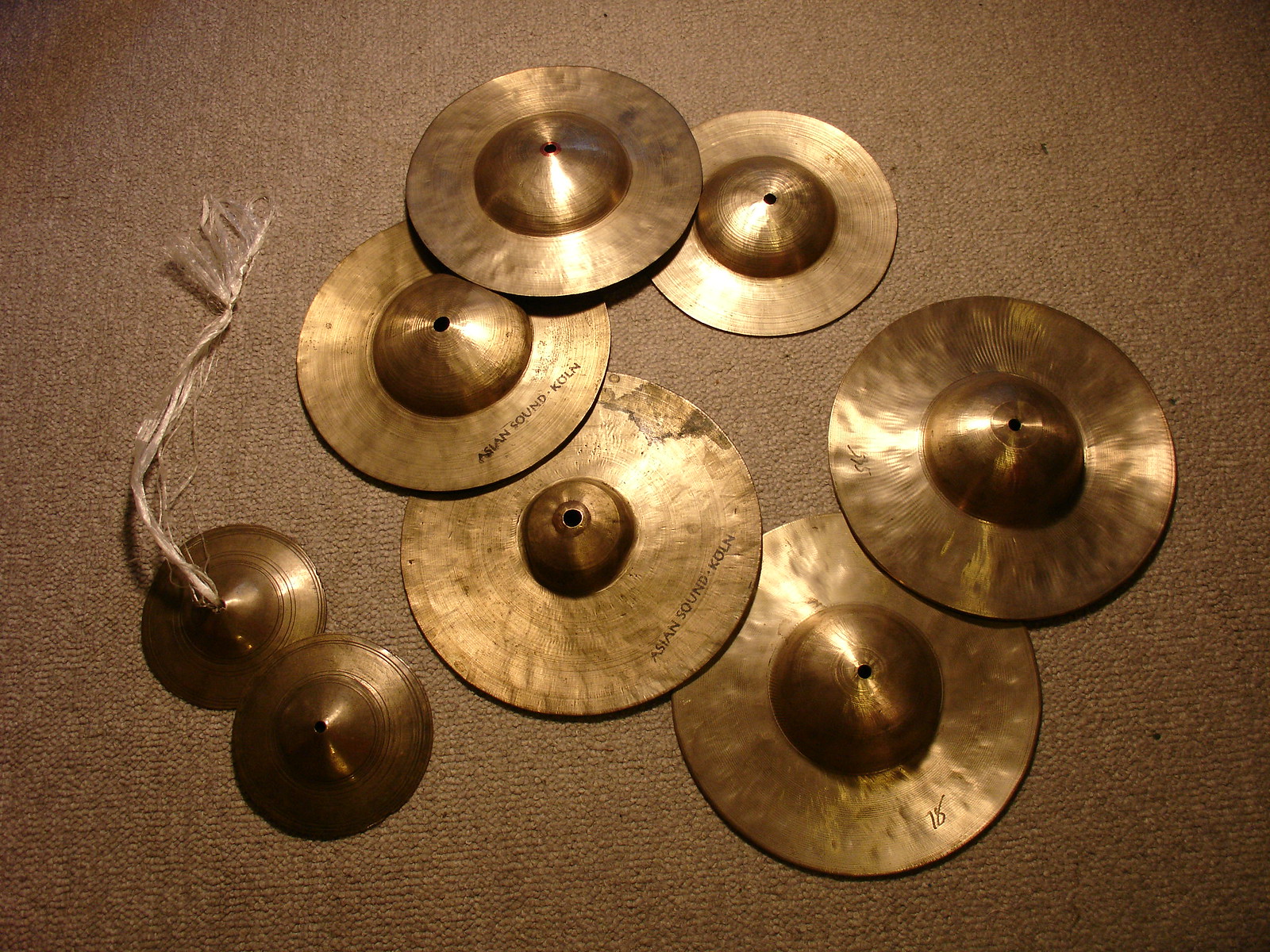The photograph depicts a collection of brass discs resembling finger cymbals, arranged in a circular pattern of six with two additional smaller cymbals on the lower left-hand side. These discs feature a small dome in the middle, each with a hole through it. One of the smaller discs has a rope-like string threaded through its center. The cymbals exhibit some slightly rusted areas and inscriptions that read "Asian Sound" along their edges. The background is a light brown, short-pile carpet, reminiscent of a linen or cotton texture with a bronze-like hue. The overall setup and the appearance of the cymbals evoke a sound similar to that of traditional cymbals when struck or strung together.